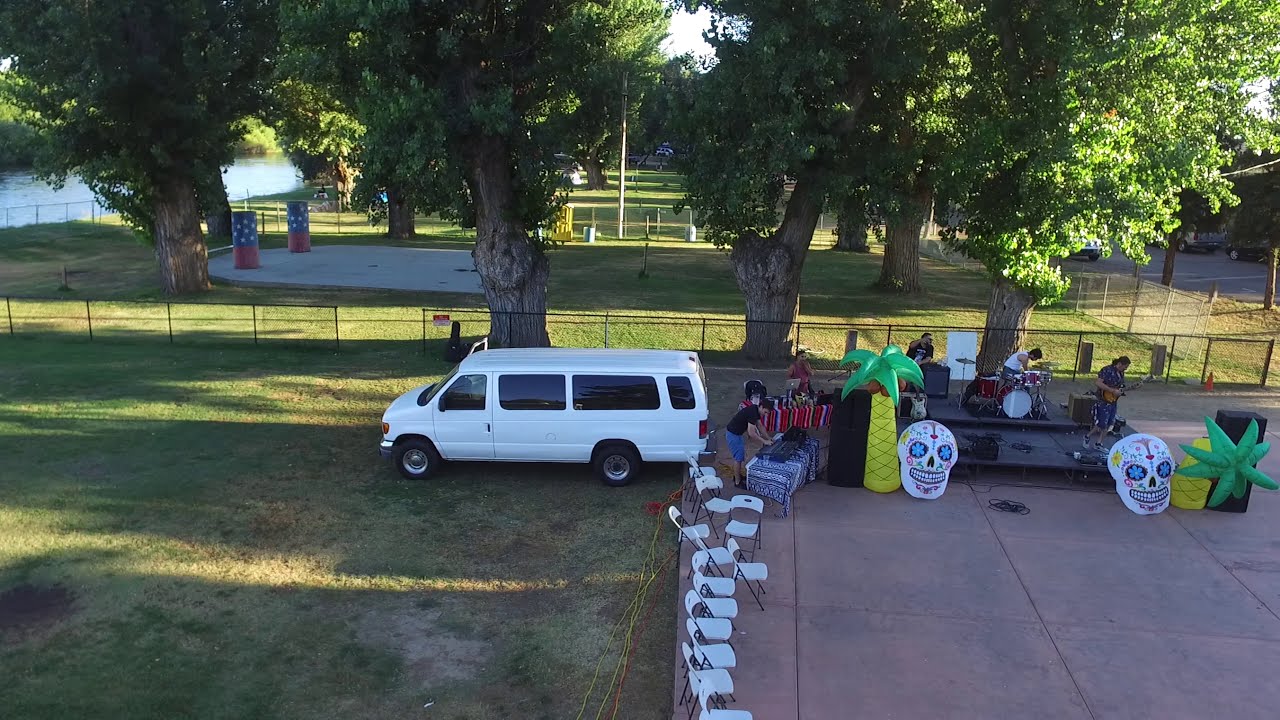The image showcases a vibrant scene in what appears to be a public park, with lush, green surroundings and thick tree trunks. Five prominent trees frame a cement area, which is covered partially by green grass. A white van is parked directly in front of this space, perhaps having transported the musical instruments and equipment. The focal point of the area features a small stage made of black plastic pallets, where several musicians are setting up — including a drummer, a guitarist, and a person working on a laptop. In front of the stage, there are inflatable palm trees and Day of the Dead decorations, such as inflatable sugar skulls, adding a festive atmosphere. A guy is seen setting up what seems to be a DJ station. To the left of the stage, there's a table being arranged, and in the foreground, a line of white chairs has been placed for the audience. The backdrop includes a fenced-in open field, tall trees, and in the far distance, a basketball court is visible. The photograph appears to be taken from an elevated viewpoint, perhaps an upper window or a roof, capturing the preparation for what looks like a Day of the Dead-themed concert event.